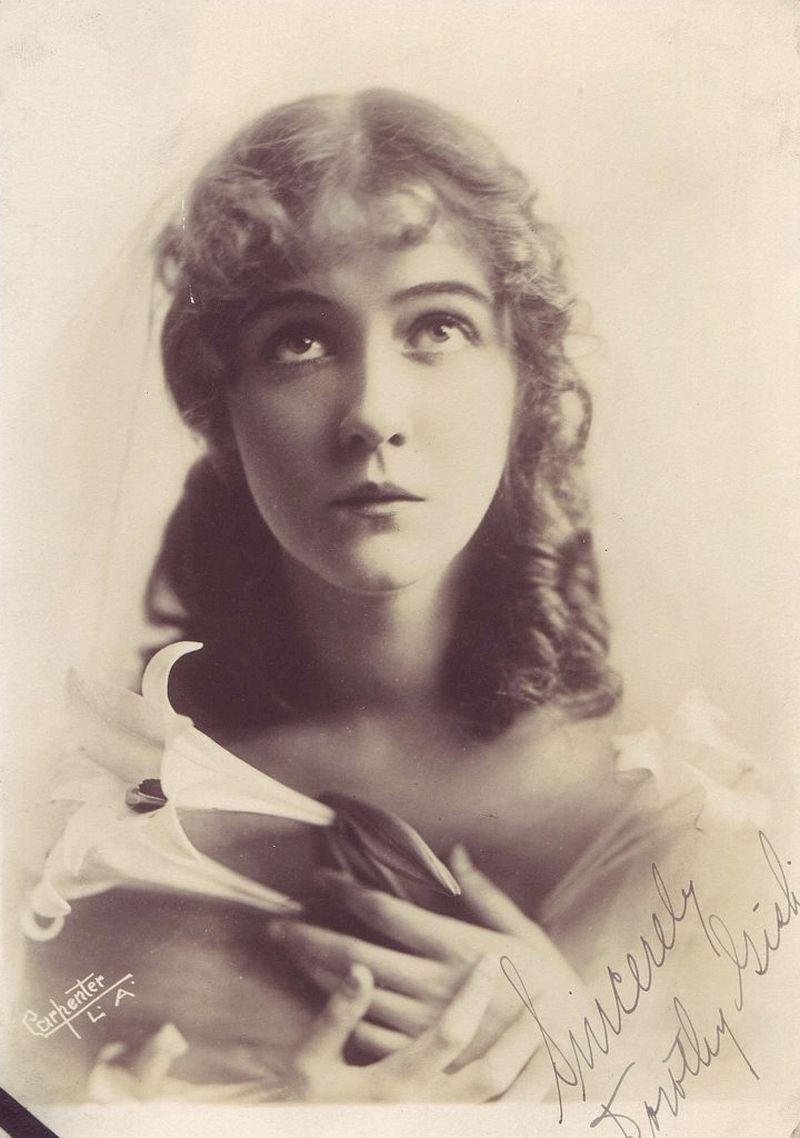This is an old black-and-white portrait of a young Caucasian woman with curly, shoulder-length brunette hair, featuring prominent curly bangs that frame her face. Her eyes are open and gazing upwards, giving the impression that she is looking towards the sky. Her lips are closed and slightly pursed. She is depicted with her hands clasped over her heart, holding two blooming white flowers in her left hand. The background of the image is a light beige color, emphasizing the vintage quality of the photograph.

At the bottom left corner of the photo, "Carhenter, L.A." is inscribed in white letters, suggesting the photographer's name and location. In the bottom right corner, there is an autograph in cursive black font that reads, "Sincerely, Dorothy," followed by a last name that appears blurry or illegible. The overall composition of the portrait exudes a nostalgic and reflective atmosphere.